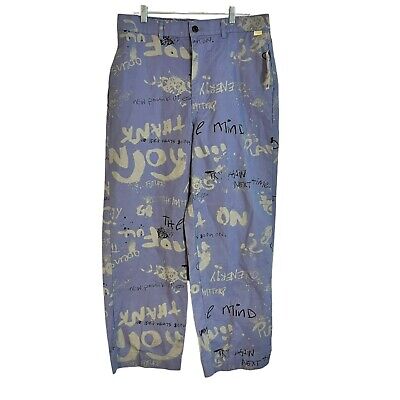This image features a pair of blue jeans, prominently displayed front and center against a white background. The jeans are hanging from a rod using two clips attached to the waistband, which includes visible belt loops and a waistband snap at the top, with a zipper below. There is a small, unreadable yellow tag just beneath the waistband on the right side. The jeans, likely designed for edgy or street fashion, are adorned with various scribbles and words in black, white, and yellow ink. Some of the discernible words include "thank you," "mind," "energy," and "enjoy," while other inscriptions are harder to make out. Creamish yellow splotches can also be seen among the writings, adding to the artistic and graffiti-like appearance of the denim. The overall color of the jeans is a light bluish gray.